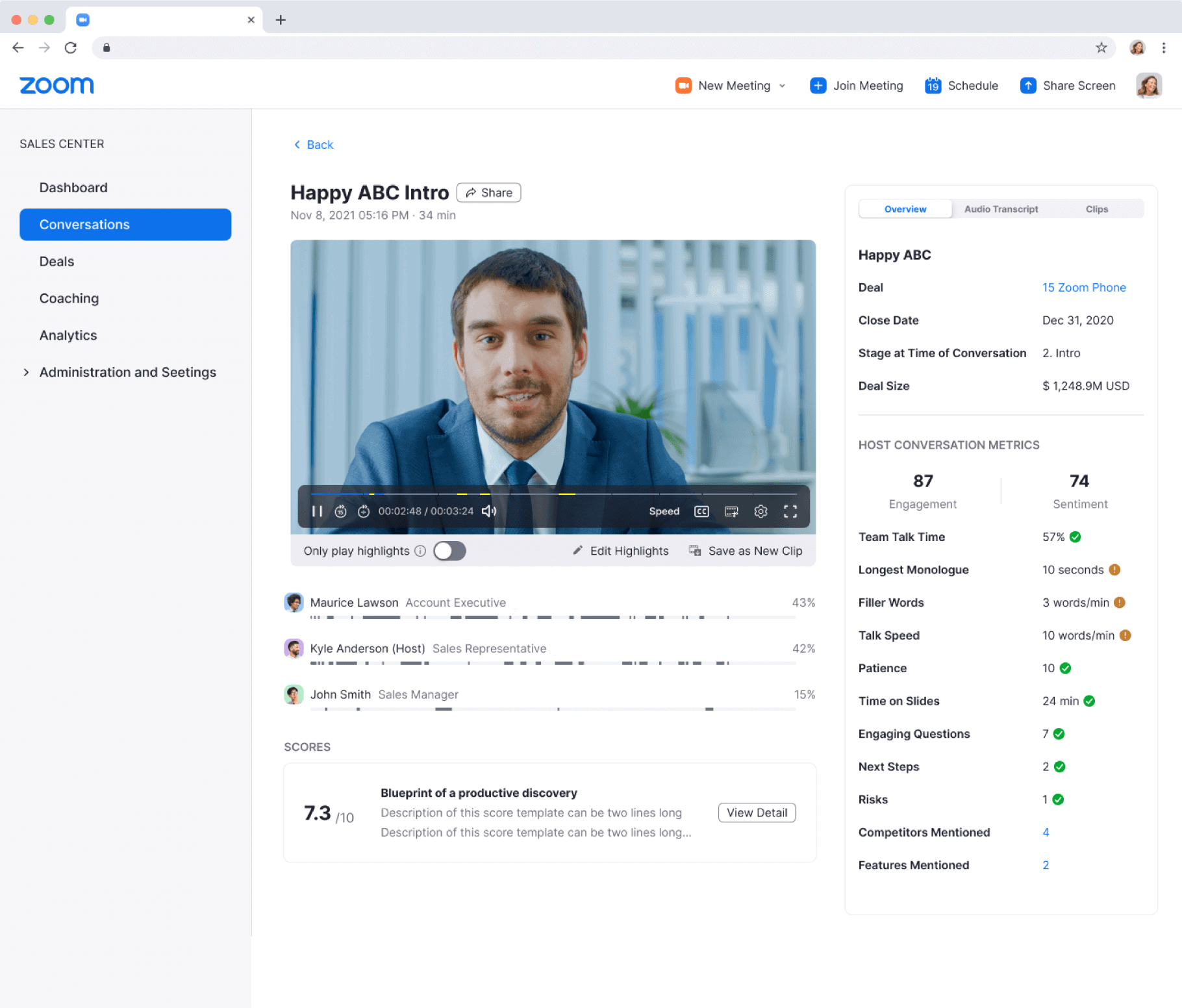This image is a detailed screenshot of a Zoom meeting interface. At the very top, the word "Zoom" is prominently displayed. The main section of the screen features a video box with a participant, who appears to be involved in the meeting, and is labeled "Happy ABC Intro". Along the right-hand side, there is a vertical panel that offers several options: Overview, Audio, Transcript, and Clips. 

Under the Overview tab, various details related to the meeting are listed, including "Happy ABC", "Deal: 15 Zoom Phone", "Closing Date", "Stage at Time of Conversation", and "Deal Size". Additionally, there is a section labeled "Host Conversation Metrics", which includes numerous analytical metrics such as Team Talk Time, Longest Monologue, Filler Words, Talk Speed, Patience, Time on Slides, Engaging Questions, Next Steps, Risks, Competitors Mentioned, and Features Mentioned.

At the bottom of the video box, a score of 7.3 is displayed alongside a label "Blueprint of a Productive Discovery". Below this, there are comments or scores from other participants, expressed in percentages, indicating their feedback or evaluations.